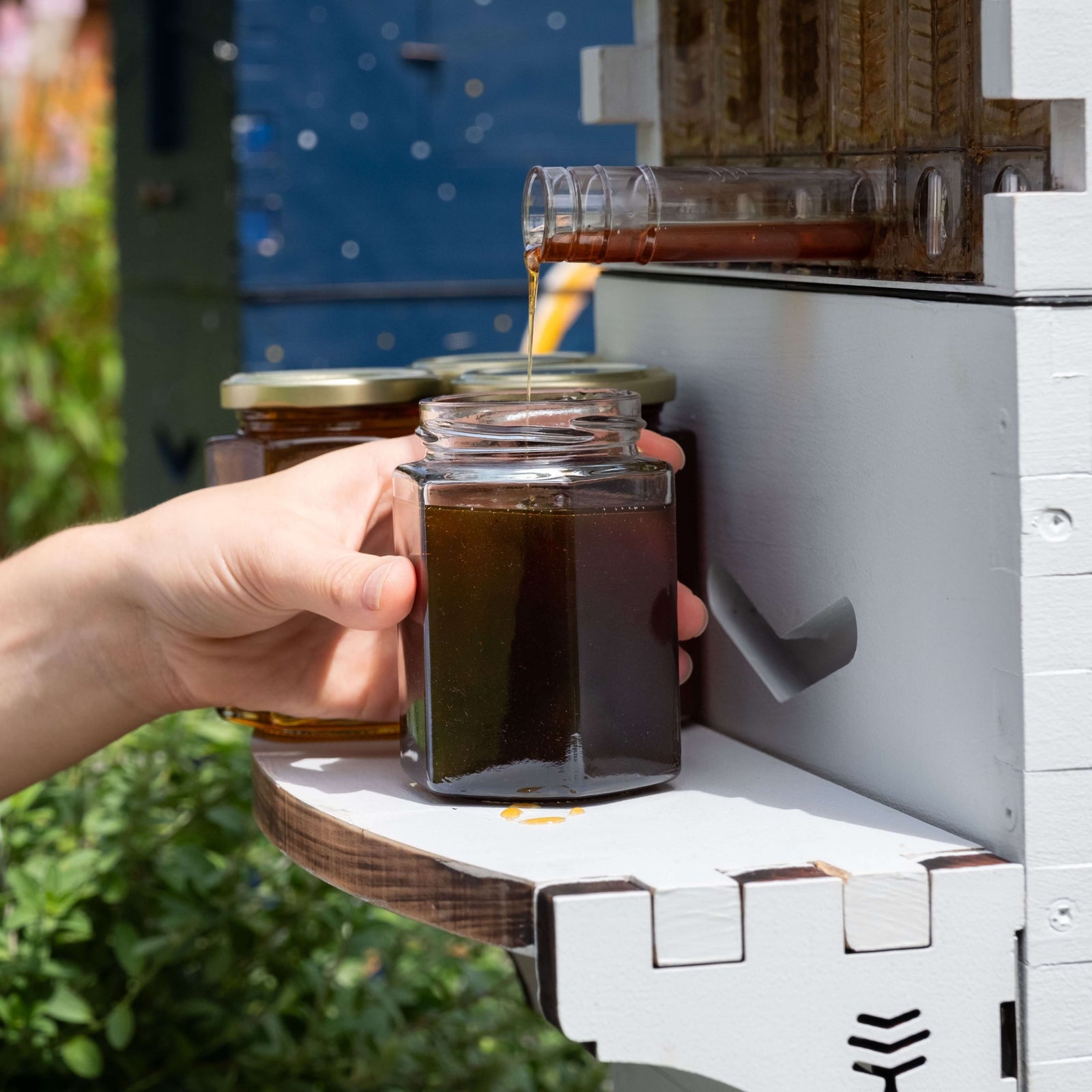The photograph captures a close-up scene of honey being harvested from a beehive. A person’s left hand is seen entering the frame from the left, holding an open, hexagonal jar underneath a plastic spout. Honey is pouring out from the spout, which emerges from a white-painted, wooden beehive. The top of the hive features multiple potential spout holes, though only one is in use, and this section is left unpainted, showing natural wood. Behind this active beehive, two other white-painted, stacked blue beehives are visible. The background features lush green foliage and small bushes, creating a natural setting. The honey-catching jar is nearly full, and several similar jars with golden lids are arranged behind it on a white shelf that is part of the beehive stand. The scene is detailed with the rich, dark honey contrasting against the pale wood and vibrant greenery.